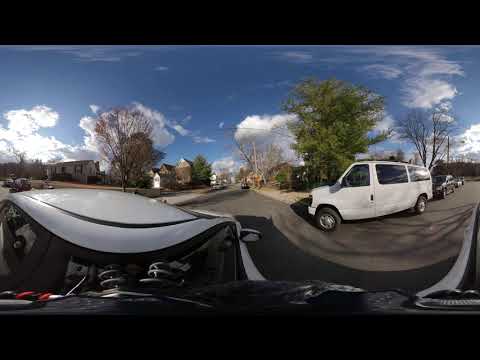The scene is a view from possibly the interior of a black-colored motorcycle or car, looking out onto a curving, slightly distorted street. On the right side of the street, a white van is in the process of turning right. Behind this van, another vehicle, possibly black, is visible, along with several other indistinct cars. The sky above is a brilliant blue, dotted with large, fluffy white clouds. 

To the right of the scene stands a big, green leafy tree, contrasting with a relatively bare tree on the left. In the background on the left side, a white house is visible, along with another, further back, reminiscent of a farm building. Additional houses with white and brown exteriors and different colored rooftops can be seen in the distant background, indicative of a residential neighborhood.

The bottom of the image reveals part of the black frame of the motorcycle or car’s interior, emphasizing the exterior view. The street features a solid white line on the right side and overhead streetlights are peppered throughout the scene. There is no text present in the image, and no people can be clearly discerned.